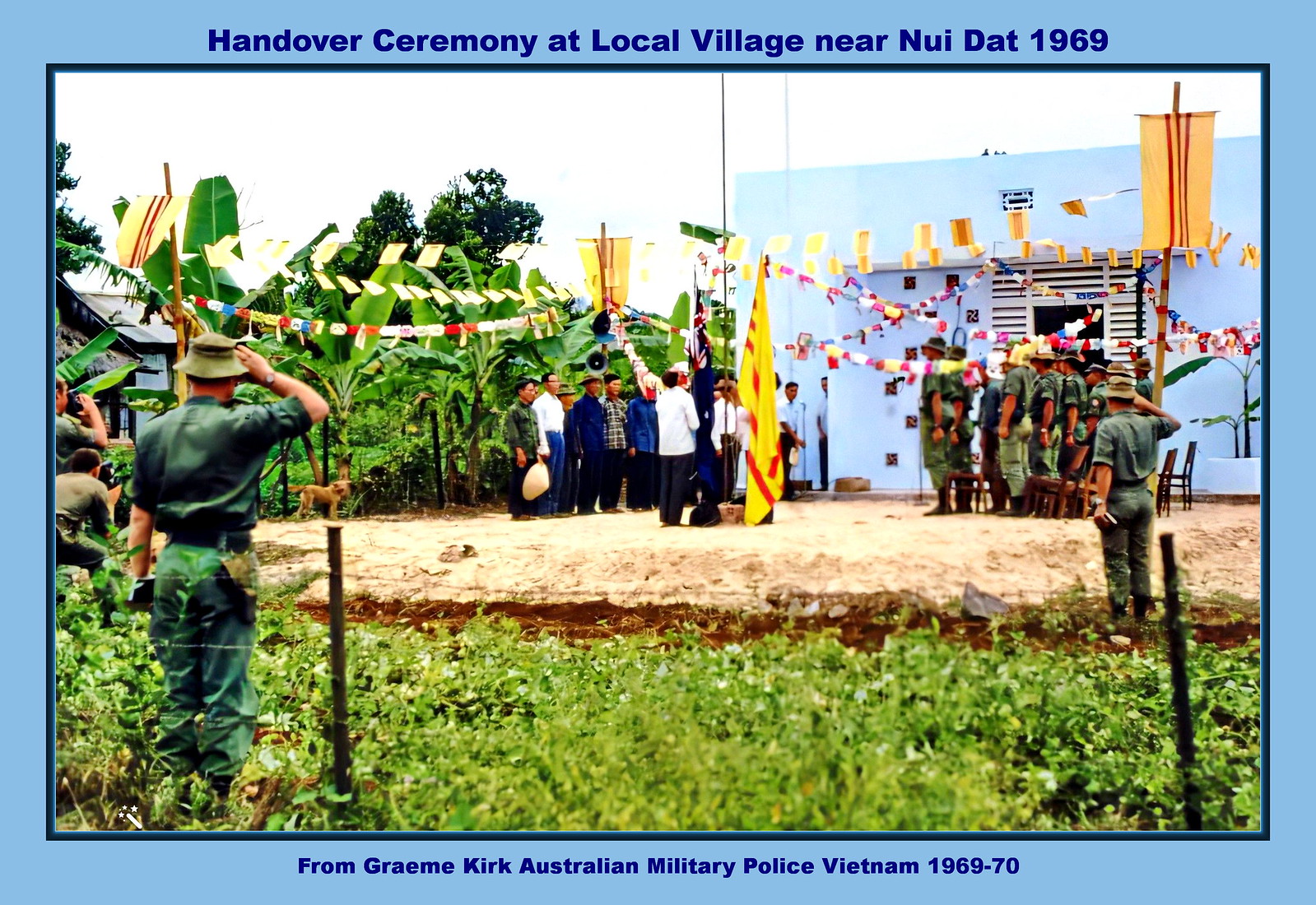The image depicts a "Handover Ceremony at a local village near NUIDAT, 1969," with a blue border surrounding it. At the top, the title is inscribed in dark blue text, and at the bottom, another blue banner reads, "From Graham Kirk, Australian Military Police, Vietnam 1969-1970." The scene shows a daytime ceremony in a lush, green area, likely in Vietnam. The foreground includes crops and a barbed wire fence. To the right, a blue building stands beside lined-up soldiers in formation. In the center, a large yellow and red flag is being handled by men flanked by military personnel on both sides. The background features abundant vegetation, possibly including banana trees and cornfields. Multiple photographers and additional people, likely local villagers, can also be seen, with soldiers in green uniforms and beige hats saluting. The sky is clear and white, adding to the serene yet formal atmosphere of the event.